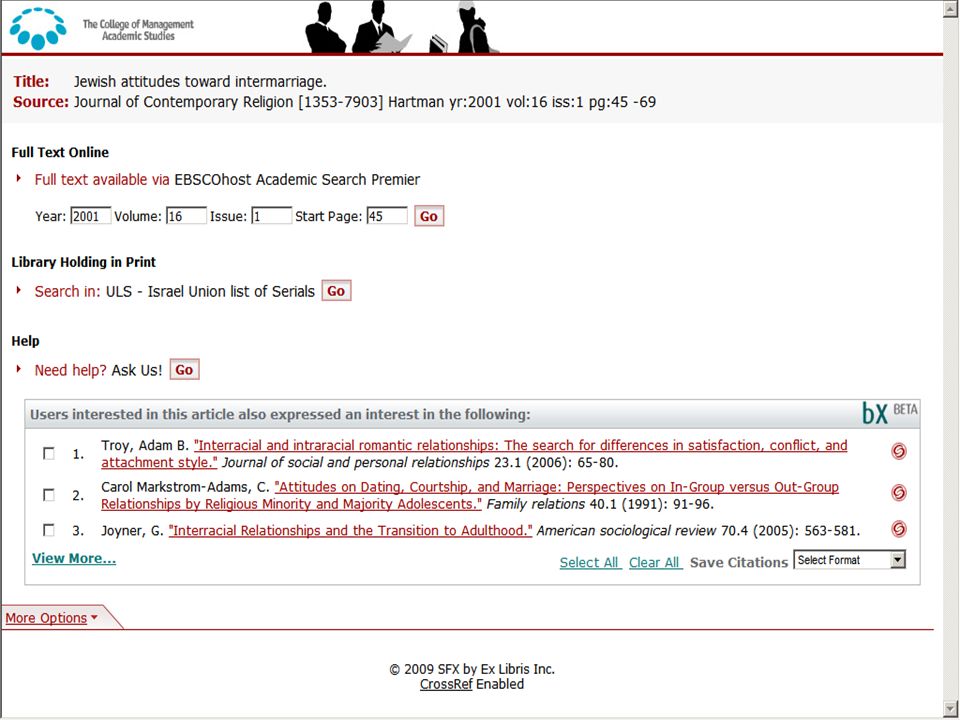This image is a detailed screenshot from an academic resource interface affiliated with the College of Management Academic Studies. In the upper left-hand corner, the screenshot highlights a specific article titled "Jewish Attitudes Toward Intermarriage," sourced from the Journal of Contemporary Religion (ISSN: 1353-7903). This article, authored by Hartmann in the year 2001, is found in Volume 16, Issue 1, spanning pages 45-69.

The interface provides multiple access options, including a link to the full text available online, accessible via EBSCO Host Academic Search Premiere, with a direct start page at page 45. The interface also mentions library holdings in print and includes a search option in the ULS Israel Union List of Serials.

Additionally, there is a "Help" section offering assistance, and the interface notes that users interested in this article often show interest in three other articles, each listed with the respective author, title, and a notable quote.

At the bottom center of the screenshot, the year 2009 is marked, with a note of "SFX by Xlibris Incorporation, Crossref Enabled," detailing the digital infrastructure and cross-referencing capabilities provided.